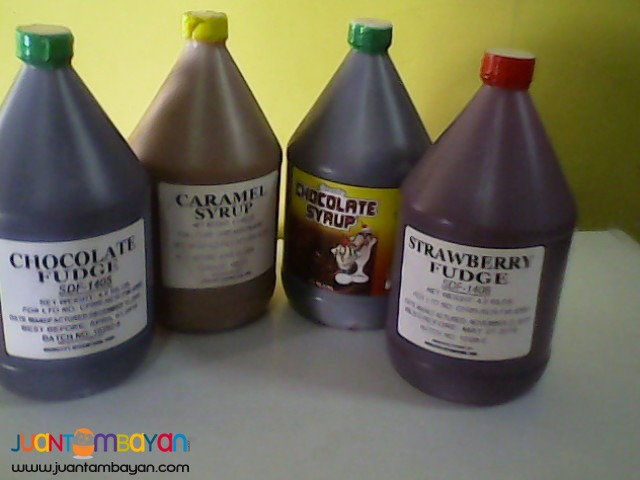The photograph, though slightly blurry, depicts a yellow wall behind a white table on which four large, transparent plastic jugs are lined up. Each jug has a distinct label and color-coded cap, indicating its contents. From left to right, the labels read: "Chocolate Fudge" with a white background and a green cap, containing a dark brown substance; "Caramel Syrup" with a yellow cap and light brown interior; "Chocolate Syrup" with a green cap, a red and brown label featuring what seems to be a cartoon image of ice cream, filled with dark brown syrup; and "Strawberry Fudge" with a red cap, containing a reddish-brown substance. Positioned at the bottom left of the image is a logo and URL that reads "Juan T. Mabayan, www.juantmabayan.com." This collection of jugs, likely used for dessert toppings, demonstrates the importance of labeling to differentiate the liquid contents, which could otherwise be mistaken for non-edible substances due to their generic packaging.